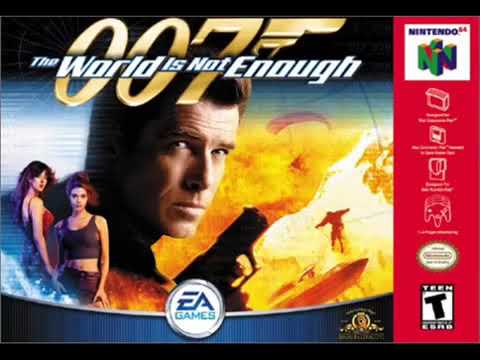The image is the cover of a Nintendo 64 game titled "007: The World is Not Enough." Dominating the top center in gold is the iconic "007" logo, featuring a small golden gun next to it, signifying James Bond’s license to kill. Superimposed on this logo is the movie's title, "The World is Not Enough," in white text.

Central to the cover is a striking image of Pierce Brosnan as James Bond, staring intently at the viewer, while holding a black revolver. Surrounding him, particularly to his left, are two women: one with long brown hair wearing a red bra, and the other with her hair in a bun, dressed in a black spaghetti-strap top, suggestive of their roles in the film.

The background is a dynamic montage: to the right is a blend of fiery explosions and distant figures, contributing to the action-packed theme. The bottom center features the EA Games logo, while an MGM symbol is positioned nearby.

Along the right edge is a bold red vertical stripe. At its top is the word "Nintendo," identifying the platform, followed by the Nintendo 64 emblem with two green letters "N." Below this segment are additional details about platform compatibility and ratings, including a "T" for Teen symbol within a small black-and-white square at the bottom.

This vivid and detailed cover art encapsulates the thrilling essence of the James Bond film adapted for a Nintendo 64 game.